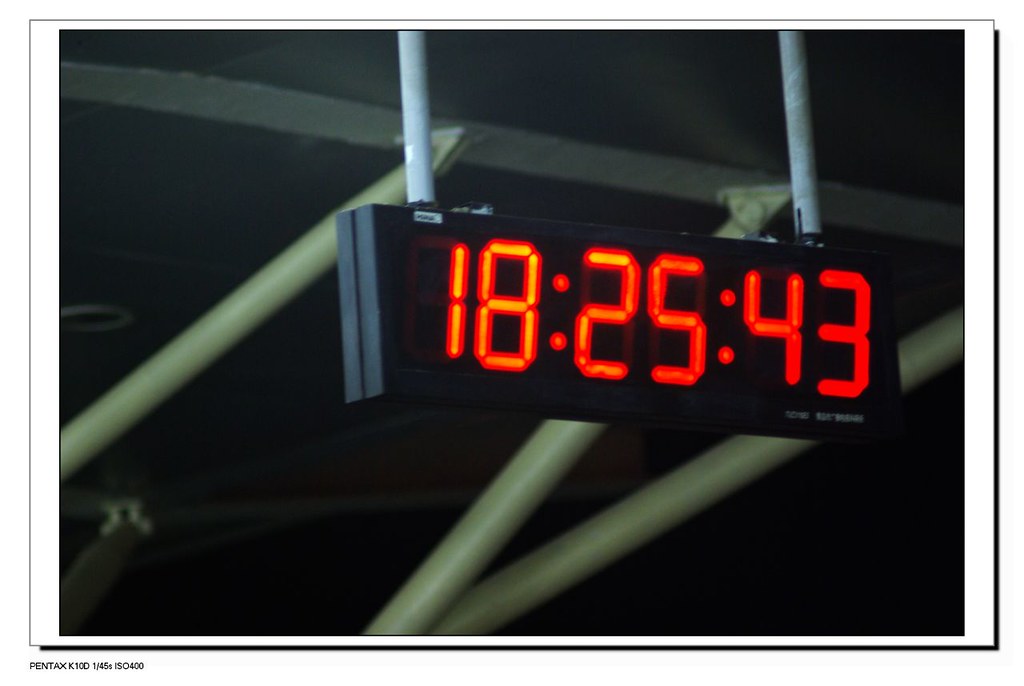The photograph captures a scene in a very dark room, making it challenging to discern specific details. The image is presented in a rectangular white frame, with a tiny, unreadable black watermark on one corner. Dominating the center of the photo is a black digital LCD clock, prominently displaying the numbers "18:25:43" in bright reddish-orange digital font. This clock, which could be reminiscent of a stopwatch, is mounted on two silver metal bars suspended from what appears to be a warehouse-style ceiling. The metal ceiling beams are a light, almost white color, and although the darkness obscures much of the background, there are hints of a black or dark gray ceiling piece and possibly a blurry ceiling fan. The scene evokes the feeling of being inside a gymnasium or similar large space, with its industrial elements and sparse, shadowy ambiance.